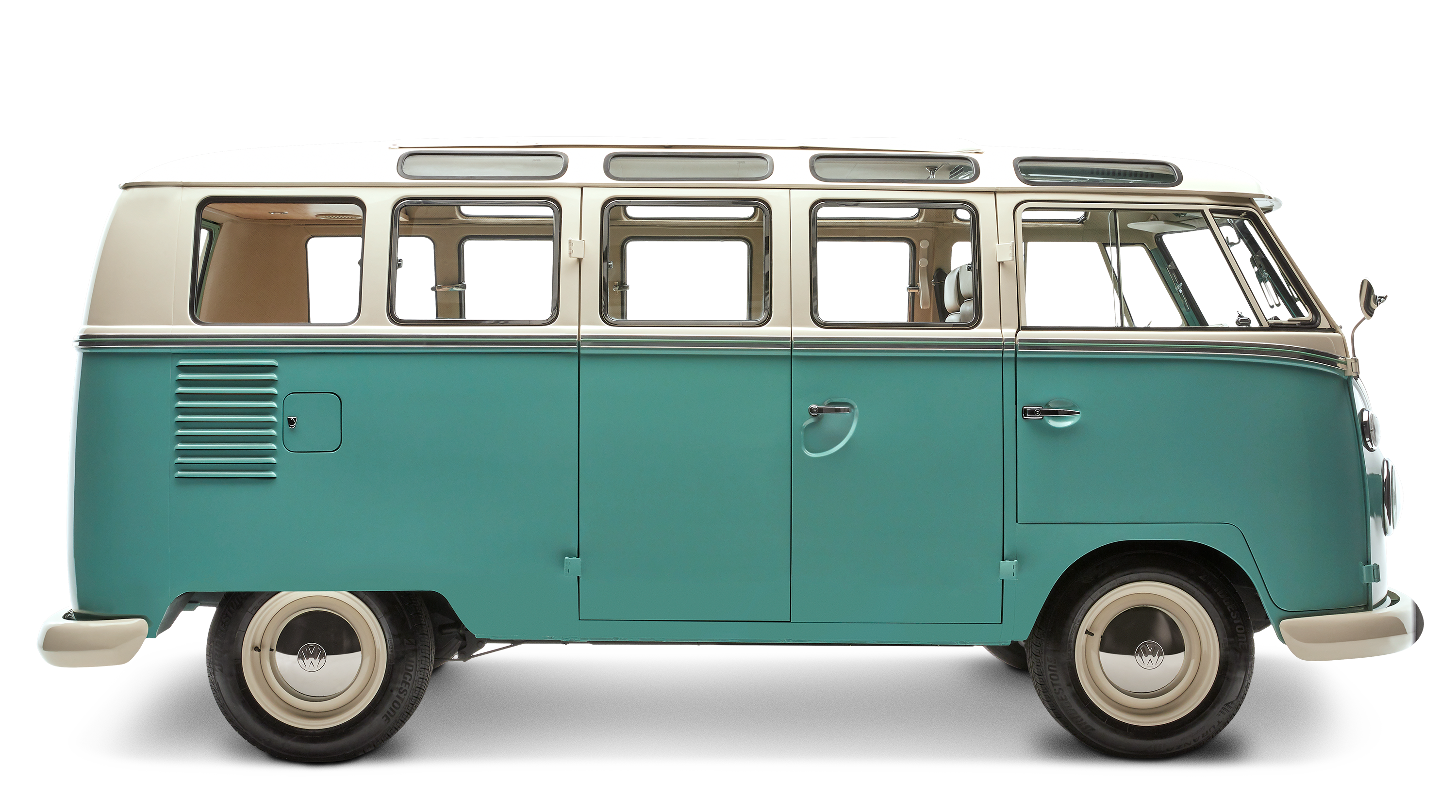This image depicts a vintage Volkswagen van, reminiscent of models from the 1950s to the 1980s, often associated with iconic media like Scooby-Doo. The van features a distinctive two-tone paint job, with a white upper half and a turquoise, Tiffany blue lower half. The design includes a unique front door and side double doors that open outward rather than sliding, akin to house doors. There are a total of ten windows along each side, including smaller windows above the main ones, as well as a front and rear window. The van is equipped with shiny silver rims, possibly emblazoned with the VW logo, matching the silver door handles. It is a multi-seater vehicle, capable of transporting up to ten passengers and exudes a nostalgic charm from its era.